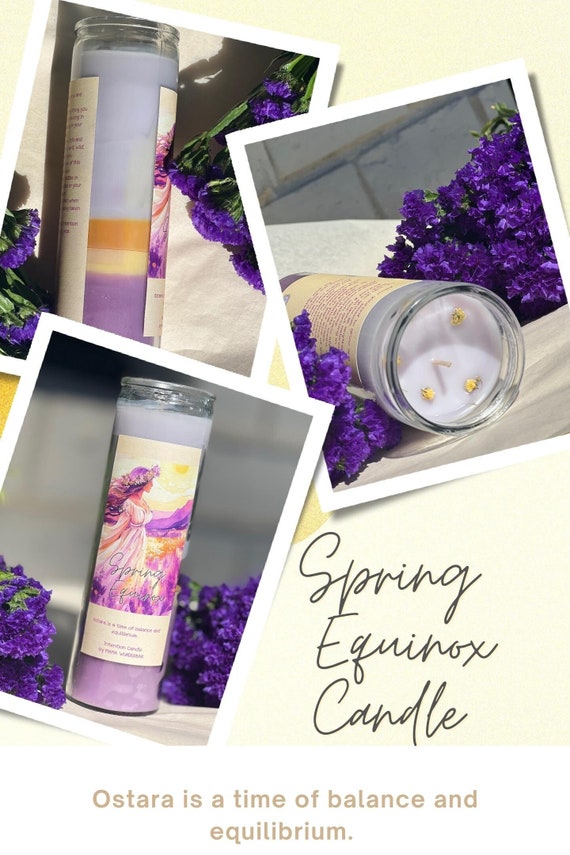The image is an advertisement for the Spring Equinox candle, characterized by its elegant and vibrant design. The main composition consists of three polaroid-style photos showcasing the candle from different angles. The candle itself is housed in a glass jar with a gradient color scheme that transitions from a deep purple base, through yellow and orange, to a light gray top. Adorning the scene are bright purple flowers, set against a light gray background, enhancing the spring-like ambiance.

One photo shows the candle upright, highlighting its tiered color layers. Another photo displays the candle on its side, offering a clear view of the wax and wick from above. The final photo focuses on the candle's label, which features a young woman with flowy purplish hair, a light lavender dress, and an atmospheric scene of a sunset over purple mountains. The candle's name, "Spring Equinox," is written in cursive black letters on the label, while beneath it in beige letters, the phrase "Ostara is a time of balance and equilibrium" further emphasizes the theme of harmony and renewal.